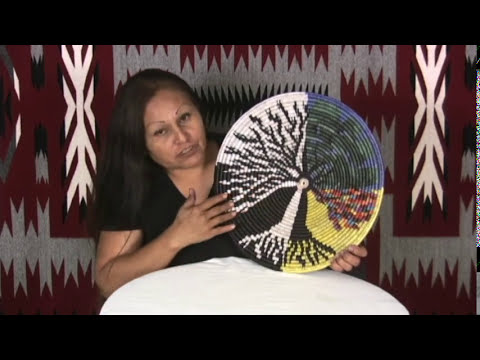In this color photograph, a woman with shoulder-length, straight black hair is displaying a round, intricately crafted object. She appears to be just shy of middle age, wearing a black t-shirt. The object she holds is an embroidered piece of art that depicts a tree with roots and branches, segmented into four quadrants. Each quadrant features a distinct color scheme: the lower left has a black background with white tree parts, the upper left has a white background with black tree parts, the upper right showcases a blue background with green tree parts, and the lower right displays a yellow background with black roots and red-accented branches.

The woman is positioned slightly to the left of center, with her hand prominently showing the back as she holds the circular artwork. She is seated in front of a circular white table, of which only half is visible. Behind her, there is a decorative backdrop featuring a dark red and white geometric pattern that resembles a Native American design, with jagged red shapes and white arrow-like forms. The overall scene is framed by black bands at the top and bottom of the image, enhancing the focus on the central subject and her remarkable craft.